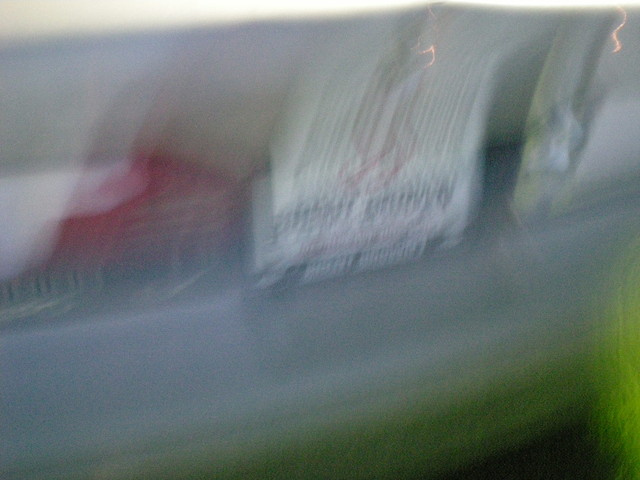This image is a blurry, underexposed rectangular frame. Its width exceeds its height. The lower right corner shows a patch of black, directly adjacent to a horizontal green strip. Above the green band, a thicker horizontal band in varying shades of blue dominates the scene. Centered, and extending upward, is a potential printed label, marred by black streaks and possibly upside-down text. The upper left corner features a hint of red, while the image's top edge reveals a light reflection, suggesting we might be viewing the edge of an object. The overall quality and ambiguity hint that this might be an AI-generated image or a photograph, but its exact nature remains uncertain.